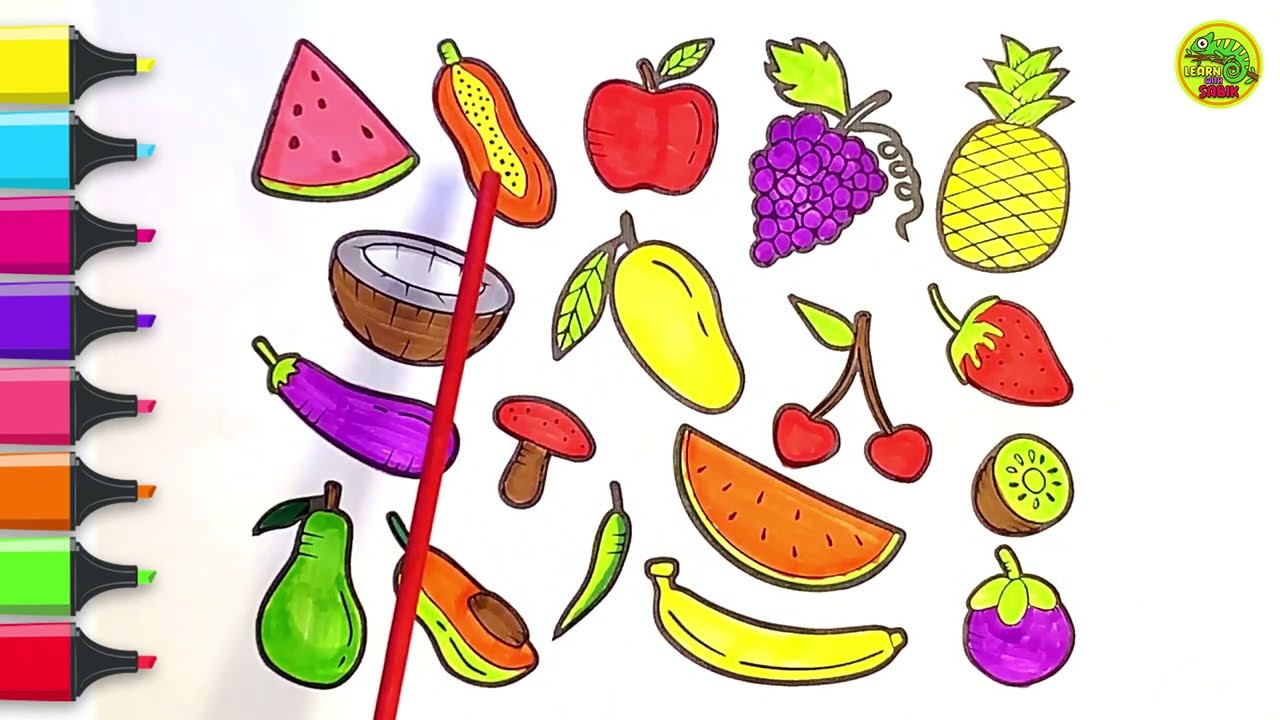The image showcases a colorful array of cartoon-style fruits and vegetables, meticulously colored with markers against a white or light blue background. On the left side of the image, eight differently colored markers are organized vertically: yellow, blue, dark pink, purple, lighter pink, orange, neon green, and red, each with black tips visible. Accompanying this are illustrations of various fruits and vegetables, vividly colored to appear almost lifelike. These include a red apple, green grapes, yellow pineapple, red strawberries, cherries, yellow squash, brown and white coconut, purple eggplant with a blue leaf, brown and red mushroom, orange fruit, green kiwi, purple plum, yellow banana, green pear, and a chili pepper. Notably, the avocado is cut in half, displaying its brown core and green-orange flesh. On the top right of the image, a logo featuring a green chameleon on a brown branch with the text "Learn with Sobik" is visible, adding an educational touch. The image, resembling a page from a coloring book, effectively captures the vibrant use of markers for artistic coloring, potentially promoting the markers themselves.